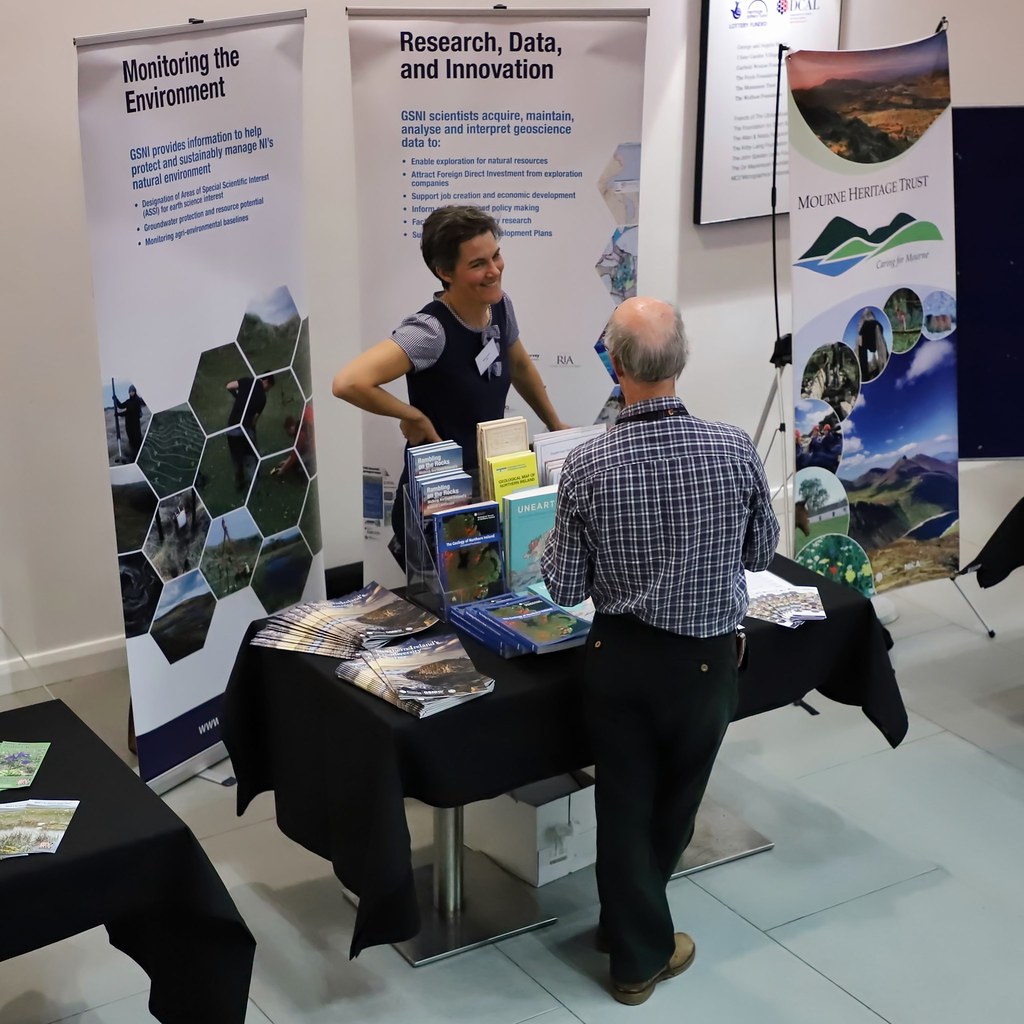In the image, we see an indoor setting with a tile floor, possibly within a museum or educational area, brightly illuminated by overhead lights. The central focus is a scene involving an elderly bald man with fringe hair, dressed in a blue checkered shirt, black dress pants, and brown shoes. He stands with one foot crossed, facing a woman who wears a jumper and a blue-toned blouse. They are engaged in discussion at a table covered with a black tablecloth, which is laden with a variety of pamphlets, booklets, magazines, and promotional materials, including fanned-out booklets, larger blue books, and a standing holder filled with smaller publications. 

Surrounding the table are several informational stand-up banners and posters belonging to the Morn Heritage Trust. These posters display key themes such as "Monitoring the Environment," "Research Data and Innovation," and other scientific and geoscience-related topics. To the right-hand side and directly behind the woman, multiple banners provide additional details, although some text is too small to read. The backdrop includes other tables and displays, suggesting that this scene is part of a larger conference or trade show exhibit, where multiple exhibits are featured. The colors in the scene range broadly, including white, black, blue, green, yellow, tan, and brown, all contributing to a professional and educational ambiance.